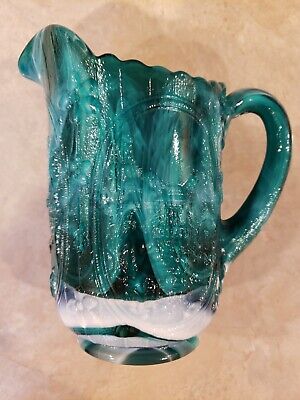This detailed photograph showcases a green mug crafted in a style reminiscent of stained glass, featuring a mixture of materials that lend it a slightly shiny and varied appearance. The mug predominantly displays green glass interspersed with other colors, creating a unique marbled effect. The mid-section and handle exhibit teal and dark gray tones, while the lower part transitions into a milky white, accented with light gray edges, giving it a translucent, marbleized look. Notably, the mug has an intricately engraved handle, matching the rest of its body in color. The background of the image is a light tan, providing a neutral backdrop that enhances the mug's distinctive hues and textures, with hints of grayish light purple adding subtle depth. The photograph is devoid of any identifying information such as time, date, or location.